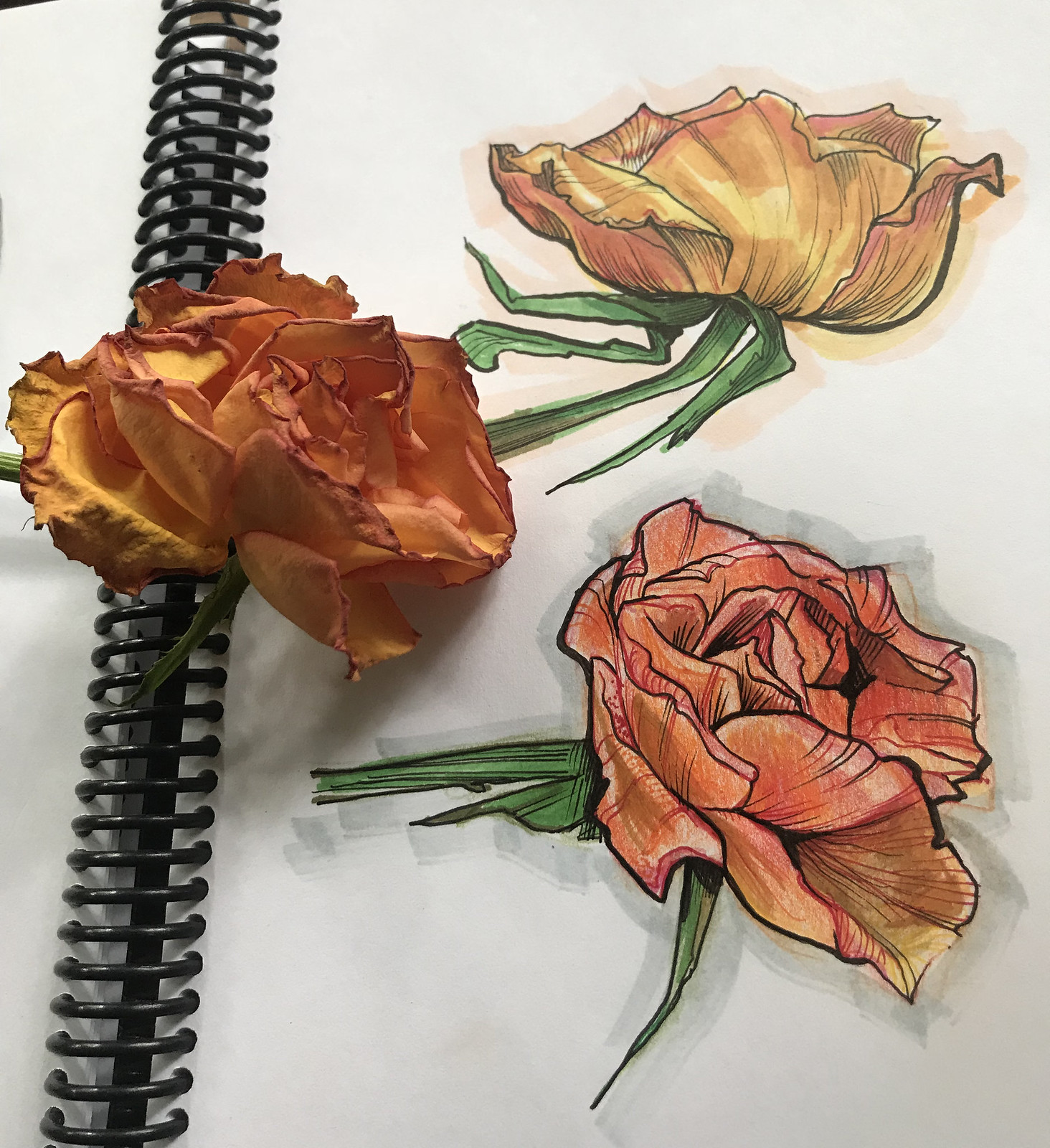Displayed on the screen is an image of an open notebook with spiral binding, revealing a beautifully detailed drawing on the right-hand page. The artwork features two striking roses. The upper rose boasts a vibrant blend of yellow, gold, and red hues. It is depicted with a green stem adorned with three leaves, detailed with black lines to emphasize the natural creases and separations. Below it, the second rose captivates with its multifaceted colors, combining shades of red, pink, orange, and yellow. This rose also has a green stem, accompanied by two green leaves positioned beneath the bloom, indicative of the supportive leaves that unfurl as the flower blossoms. A delicate gray shading behind the lower rose hints at its shadow, adding depth to the illustration. Intriguingly, beside the more orange-toned rose lies an actual orange rose, and the resemblance between the two is nothing short of stunning, showcasing an impressive and lifelike representation of the flower’s beauty.